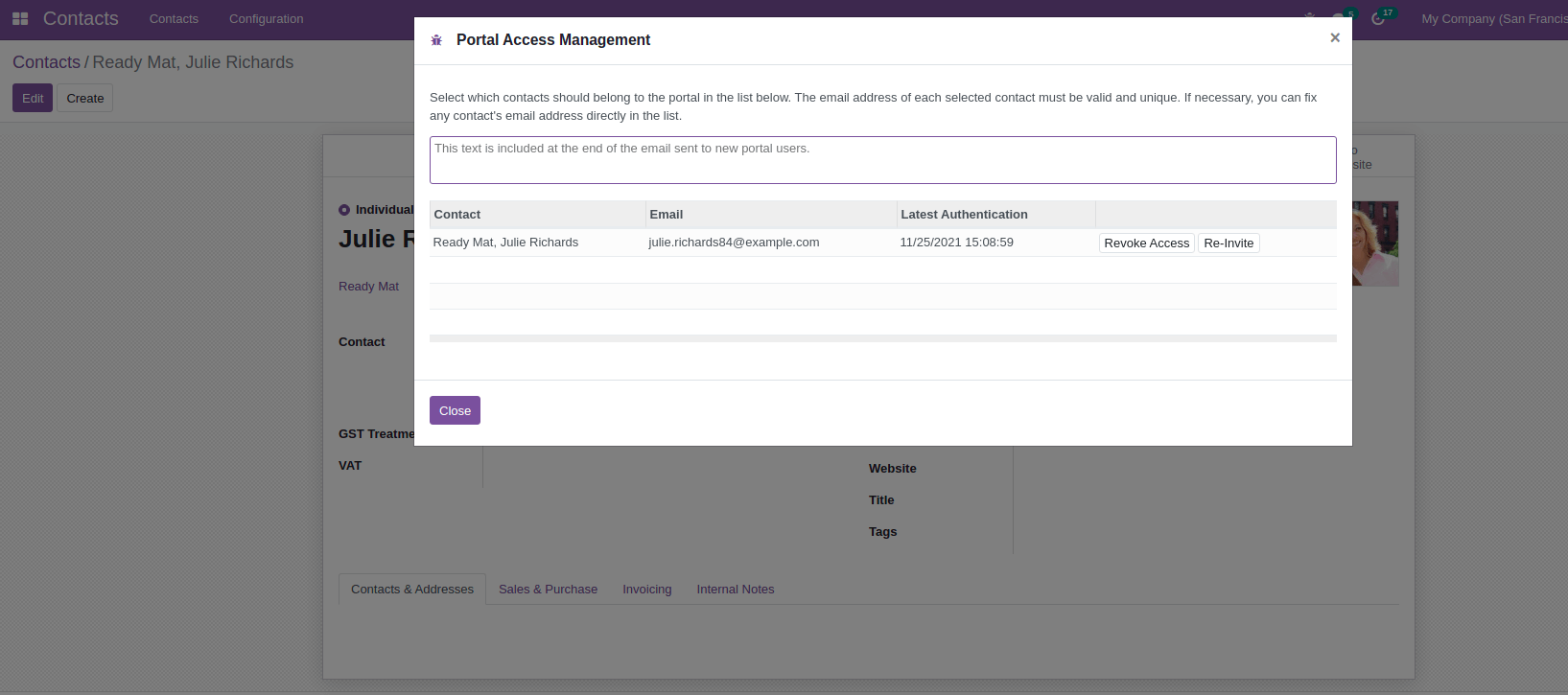In the foreground of the image, there is a prominent white pop-up window, highlighting the "Portal Access Management" interface. At the very top of this window, the title reads "Portal Access Management." Below this, there is an instructional text indicating, "Select Which Contacts should belong to the portal in the list below. The email address of each selected contact must be valid and unique. If necessary, you can fix any contact's email directly in the list."

Within this window, there is a large white text input section bordered in purple, featuring the text, "This text is included at the end of the email sent to new portal users." Farther down, a table with columns labeled "Contact," "Email," and "Latest Authentication" appears. Listed under "Contact" are the names: Ready, Matt, and Julie Richards. Corresponding emails include Julie.Richards84@example.com. The "Latest Authentication" column shows a timestamp: 12-25-2021 15:08:59.

To the right of each contact, there are two white buttons labeled "Revoke Access" and "Re-Invite." At the bottom left corner of the pop-up window, a purple button with white text labeled "Close" is prominently displayed.

In the background, the primary website is partially visible but grayed out to highlight the pop-up window. At the top of the webpage, navigation links read "Contacts, Contacts Configuration," and to the right, "My Company San Francisco." To the left side under these links, the names listed are "Contacts, Ready, Matt, Julie, Richards." Below these names are two buttons: a purple one labeled "Edit" and a white one labeled "Create." The partially visible background content appears to contain user information related to the "Portal Access Management" section.